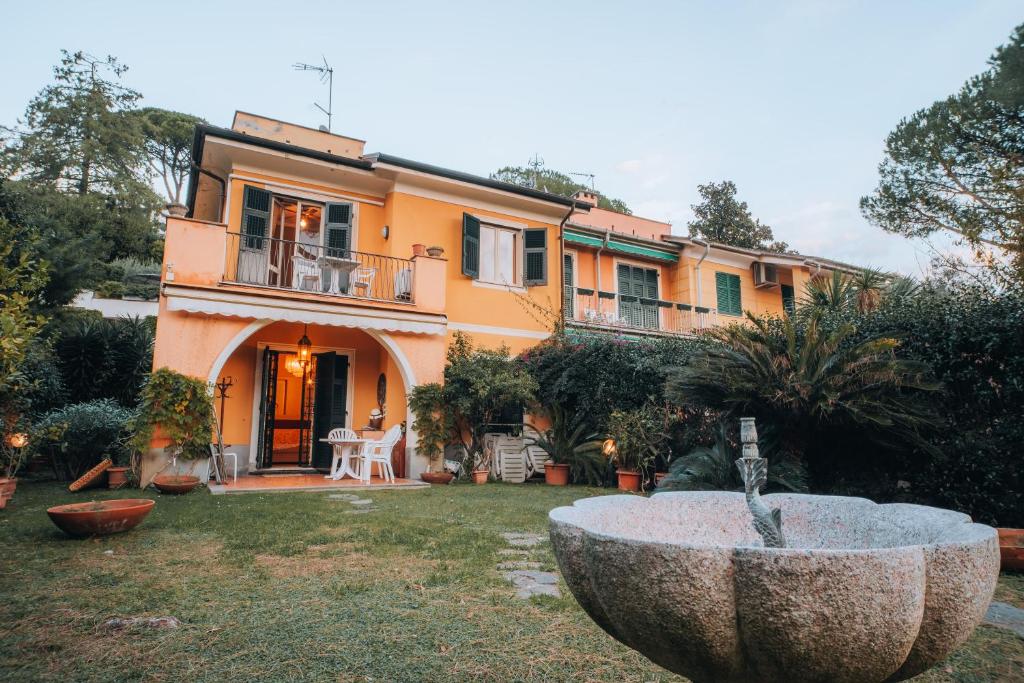The image captures a Mediterranean-style row of terraced, multi-unit villas, painted in a fading orange hue with noticeable chips and sun damage on the stucco exterior. Each two-storey house is fronted by a shabby, disrepaired garden filled with patchy grass interspersed with green, white, and brown spots. The garden is peppered with random flowered plants in flat terracotta pots arranged mostly along the edges. In the right foreground, there's a prominent stone birdbath or fountain, dry and apparently broken, with a nozzle pointing upwards.

The villas feature bi-fold doors leading to the patios and white, plastic lawn furniture on both the ground-level verandas and the wrought iron-fenced upper balconies. All windows are flanked by black plantation-style shutters, most of which are open. The top floor balconies also have similar terracotta pots as seen in the garden. The homes are lit with an orangey hue from the inside, indicating the lights are on both upstairs and downstairs. This scene suggests an evening or twilight timeframe.

To the left of the villa line stands a clump of tall trees and additional foliage, mirrored by a dense collection of bushes and plant life on the right. A TV antenna is perched atop the roofs, and further to the right, more rows of similarly coloured homes extend, their shutters closed, giving no glimpse of their interiors. The overall atmosphere conveys a quaint yet neglected charm, indicative of a long-established property teetering between cozy habitation and weathered disrepair.